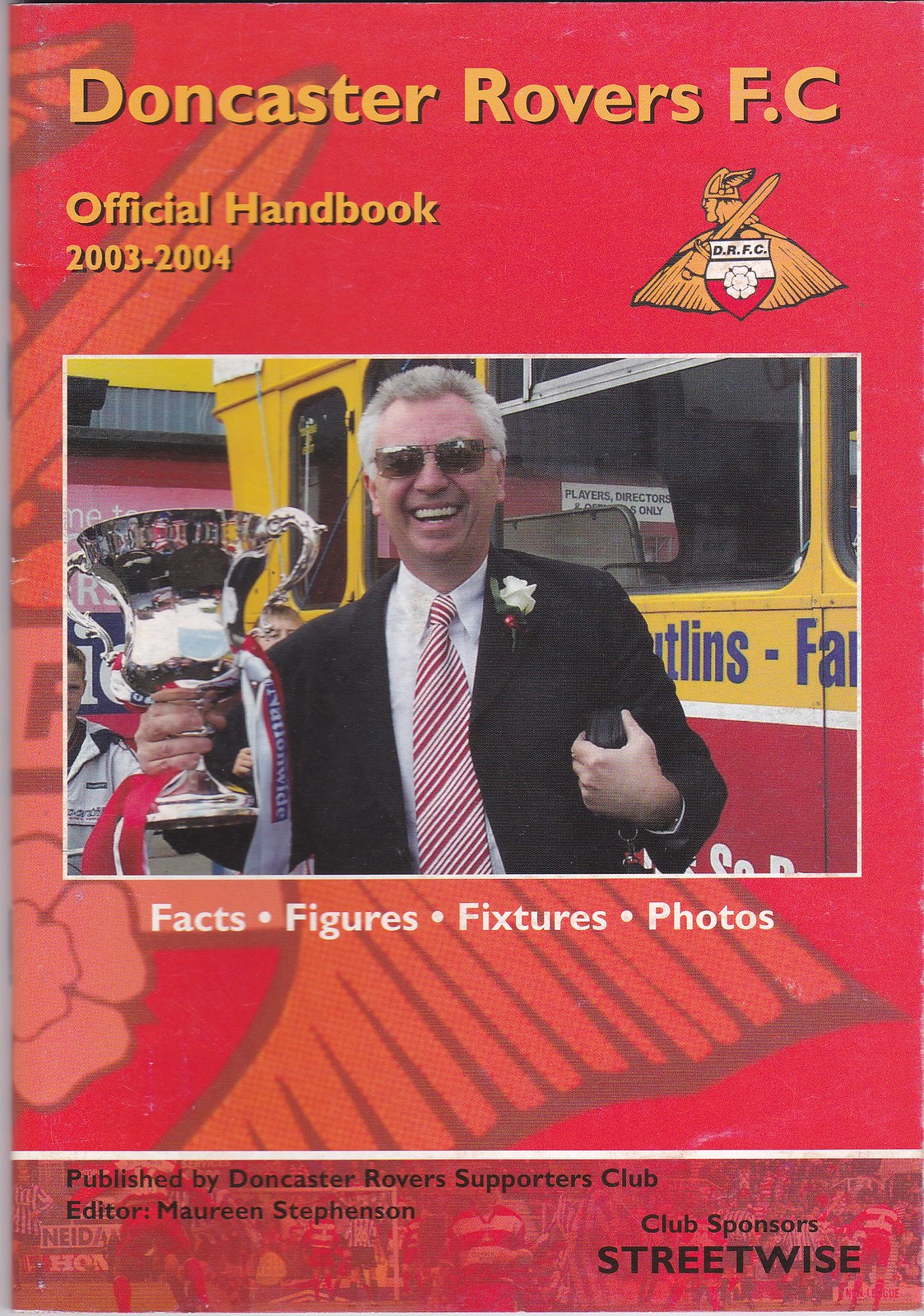The image is a color cover for the "Doncaster Rovers FC Official Handbook 2003-2004," predominantly in red with accents of orange and white. Centered is a photograph of an older man with spiky white hair and dark sunglasses, smiling. He is dressed in a black suit, a white undershirt, and a red and white striped tie. A white rose is pinned to the lapel of his suit, and he proudly holds up a large silver trophy in his right hand on the left side of the image. Behind him is a bus, and in the top right corner is the Doncaster Rovers FC logo, featuring a shield with an orange Viking. The text on the cover includes "Doncaster Rovers FC, Official Handbook 2003-2004" at the top and "Facts, Figures, Fixtures, Photos," along with "Published by Doncaster Rovers Supporters Club, Editor Maureen Stephenson" and "Club Sponsors Streetwise" at the bottom. The cover displays vibrant shades of red, orange, yellow, silver, white, and some blue, capturing the essence of the Doncaster Rovers' team spirit and heritage.